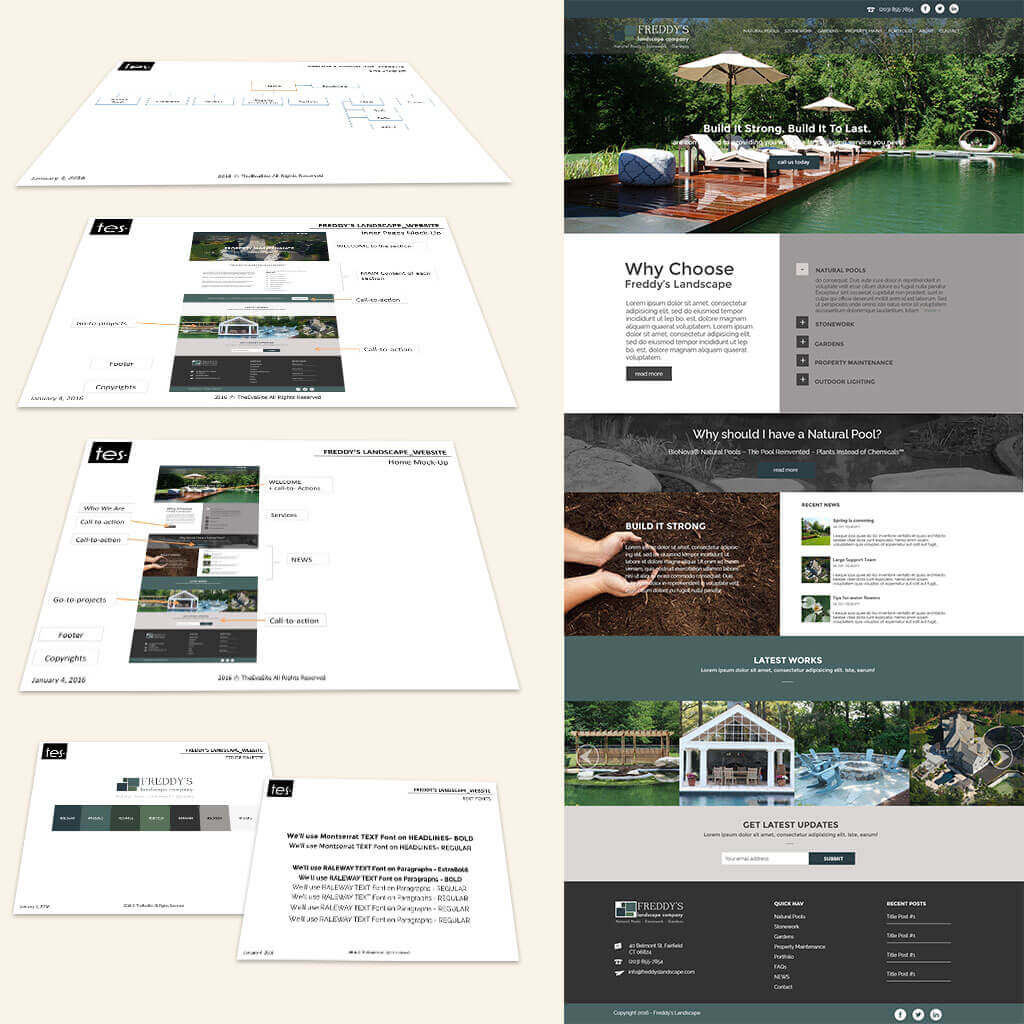This is a vertical image resembling a screenshot from a webpage. The page appears to belong to Freddy's Landscape, showcasing various sections accessible from a computer or smart device. On the left-hand side, set against a beige background, there are multiple white segments displaying blurred information. The top section features what looks like a flow chart; below it, there are blurry images apparently sourced from Freddy's Landscape website. The next segment provides a "Who We Are" blurb, followed by links to Project Services, News, and Copyrights. The bottom of this left section contains additional blurred text.

On the right-hand side, the focus remains on Freddy's Landscape. There's a section titled "Why Choose Freddy's Landscape?" featuring a descriptive blurb. Below, it discusses "Natural Pools" and their benefits. There are also options to view their latest works and updates. There is a submission bar for entering an email address to receive updates. At the bottom of this side, a dark gray box offers more clickable links, while a dark green rectangular bar holds copyright information and social media icons.